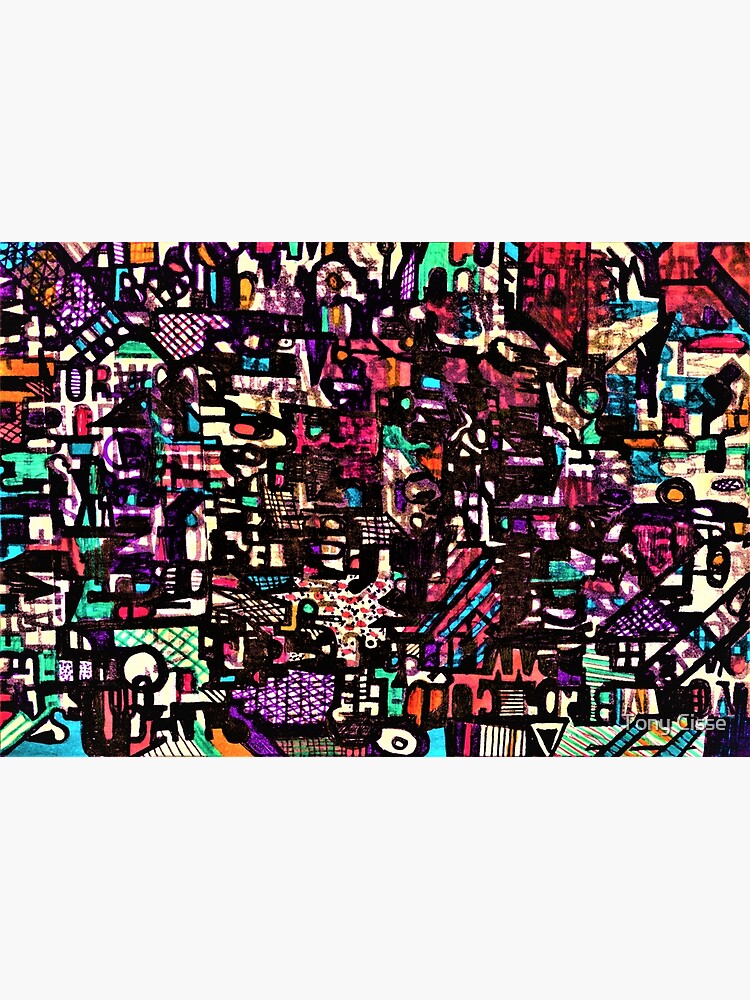This vibrant and intricate image showcases a mesmerizing array of designs and colors. Occupying the bottom 75% of the image, a stunning blend of the full color spectrum captivates the eye with an explosive palette including light blue, green, purple, black, brown, orange, white, and pink. These colors are woven into an elaborate tapestry of lines, shapes, and patterns, intertwined and layered to create a dynamic, chaotic harmony. Notably, in the bottom right corner, the name "Tony CIESE" is prominently displayed, adding a personal touch to the artwork. In contrast, the top 25% of the image is bathed in a calm light gray background, providing a serene counterbalance to the vibrant chaos below. The overall effect is a visually arresting composition that bridges colorful creativity and minimalist tranquility.